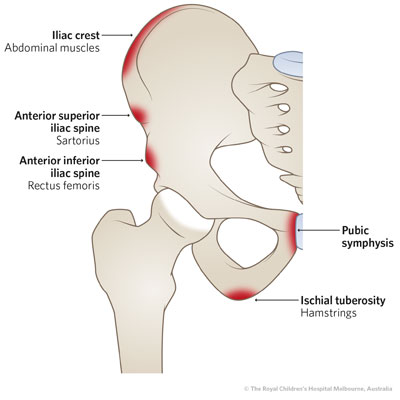The image is a detailed digital illustration depicting the right hip bone and the upper part of the connected leg bone, viewed from a perspective where the hip is on the left side of the image. The skeletal structure is colored in an eggshell white, set against a white background. Key anatomical features are highlighted in red with black text and arrows pointing to them. From the top, labels include the iliac crest, abdominal muscles, anterior superior iliac spine, and sartorius. Below these, the anterior inferior iliac spine and rectus femoris are marked. To the right, the labels indicate the pubic symphysis, and at the bottom right, the ischial tuberosity and hamstrings. These annotations suggest that the illustration is meant to serve as an educational tool, likely a medical poster commonly found in a doctor's office.